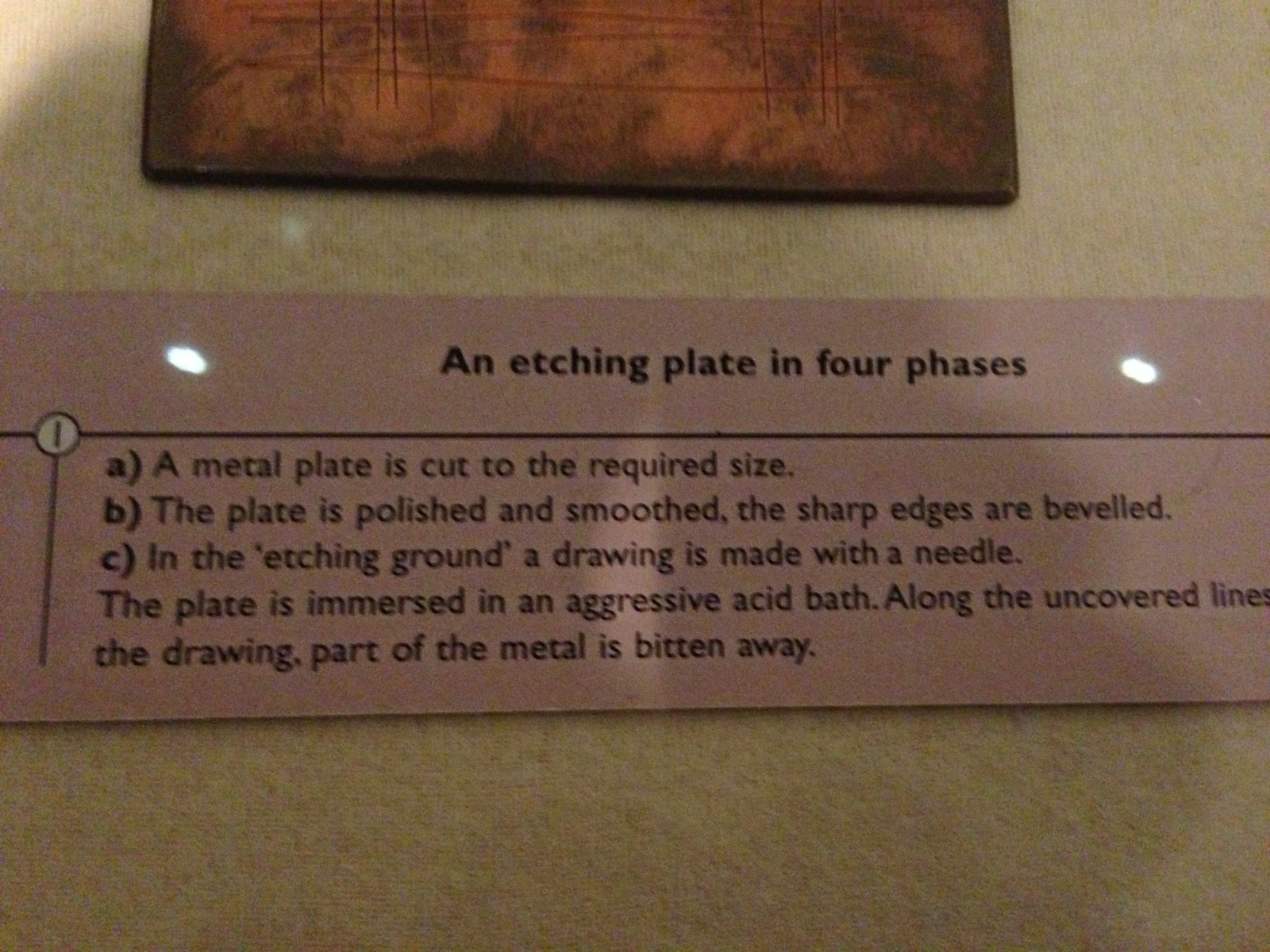This is a detailed close-up photograph of a museum exhibit sign describing an etching process. The sign, made of pink paper material with black text, is titled "An Etching Plate in Four Phases" and is positioned beneath a beige metal plate. Only the bottom portion of the artwork is visible, showcasing various tones of brown and tan with red crisscrossing lines. The plaque meticulously explains each step of the etching process: 
A. A metal plate is cut to the required size.
B. The plate is polished and the sharp edges are beveled.
C. In the etching ground, a drawing is made with a needle, and then the plate is immersed in an aggressive acid bath, causing the drawing part of the metal to be bitten away.
Additionally, there are dots of shining sunlight on the plaque, contributing to the exhibit's intricate detail.